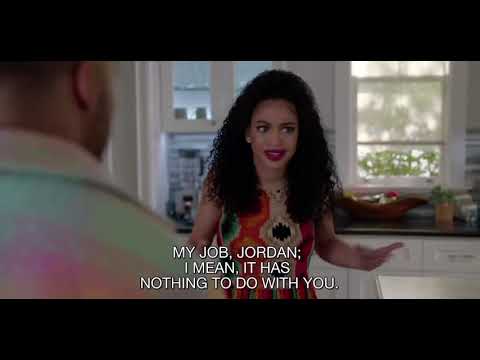The image features a scene from what appears to be a TV show or movie, framed by thick horizontal black borders on the top and bottom. Centered within these borders at the bottom are white, uppercase subtitles spread over three lines, reading: "MY JOB, JORDAN. I MEAN, IT HAS NOTHING TO DO WITH YOU." In the middle of the image is a slightly blurry black woman with thick, curly hair cascading past her shoulders. She wears red lipstick and appears to be speaking, with her mouth open and arms extended slightly outward. She is dressed in a vibrant outfit with geometric patterns in colors like orange, green, gold, and black, though it's unclear if she is wearing a dress or just a top due to the picture cutting off at her waist. She is looking towards the right. Behind her, the setting reveals a kitchen with a black countertop, scattered items, white cabinets, and a window showing some leaves outside. On the left side, the back of a man's head and neck are visible; he has some stubble and is wearing a tie-dye collared shirt with colors including blue and hot pink. He appears to be looking at the woman.